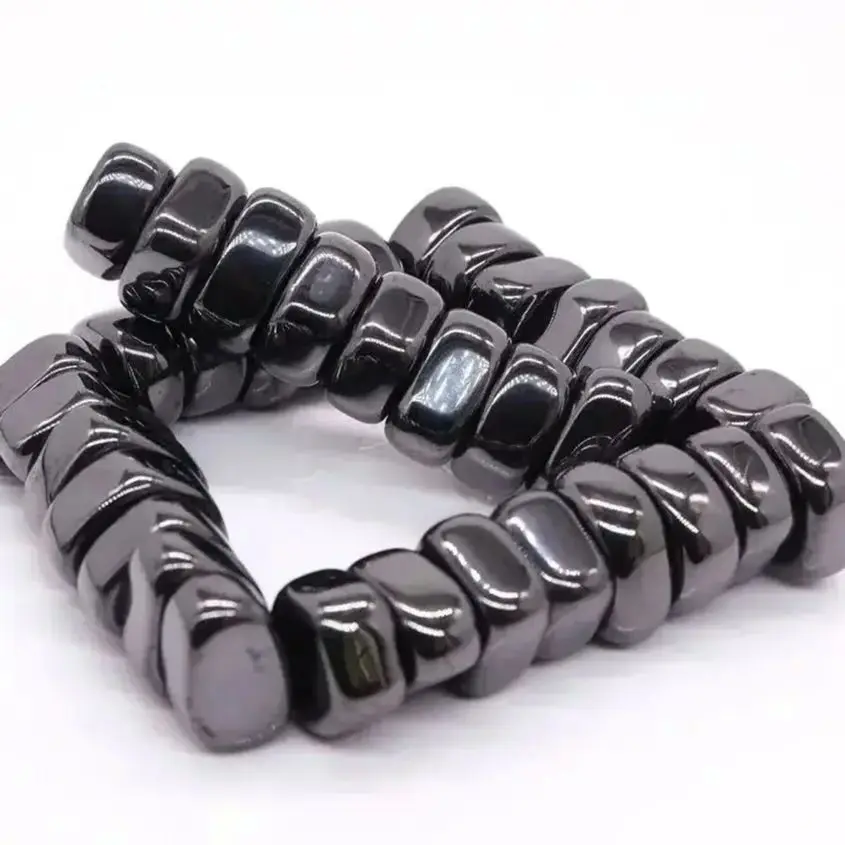This photo depicts a formation of small, naturally-shaped, oval lodestones that exhibit magnetic properties. These lodestones, appearing in shiny shades of dark gray and black, are neatly arranged against a white background. The arrangement forms a square pattern, with an additional line of stones extending from the lower right corner and ascending towards the left. Captured from a slight side angle, the stones are reminiscent of a necklace or magnetic pieces that can be detached and reconfigured. The stones, polished but varying in shape and curvature, reflect a uniform color scheme of light gray to black, suggesting a sleek, naturally-occurring texture. The photograph appears to be taken indoors.